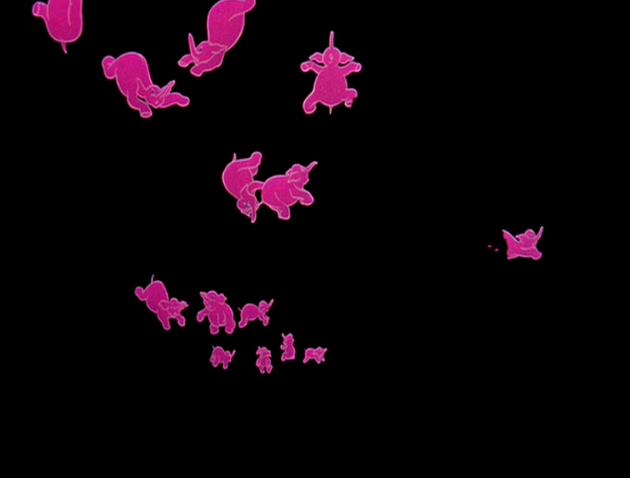This image features around 14 pink cartoon elephants set against a stark black background, creating a striking visual contrast. The elephants appear to be floating or falling through the air, each captured in various poses and scales, suggesting a dreamlike, whimsical scene. Many elephants are depicted with open mouths and wide-eyed expressions, conveying surprise or fear, which aligns with moments from the movie "Dumbo" where the titular character dreams of flying elephants. The elephants seem to be moving upwards and outwards from the picture’s center, with two or three already disappearing off the edges. Their ears and trunks are positioned differently, adding to their dynamic, cartoonish appearance. The perspective hints that the viewer is looking down at the elephants, as the ones towards the bottom of the image diminish in size, enhancing the sensation that they are falling away into the void.